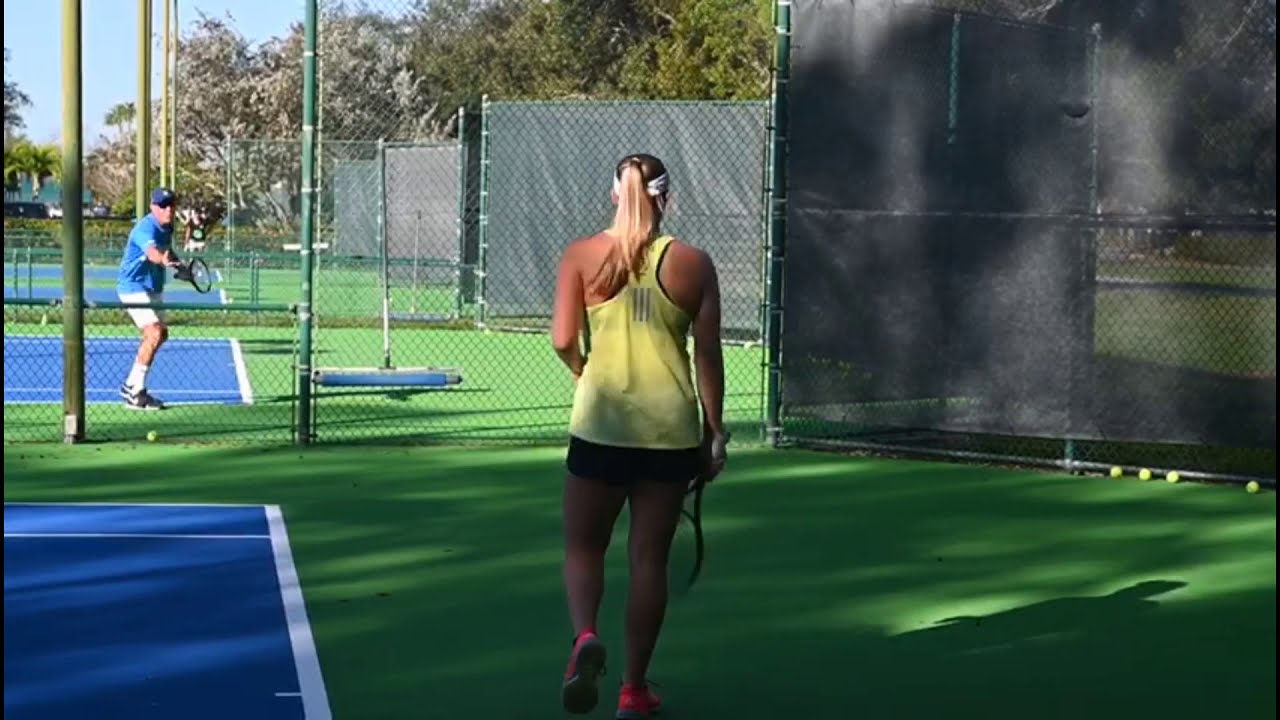The photograph captures a vibrant outdoor tennis scene on a clear, sunny day. The focal point is a tanned, blonde-haired woman, seen from behind, her hair tied back in a ponytail and adorned with a white headband. She is poised to serve, standing behind the baseline on a blue tennis court with green surrounding areas. The woman is dressed in a yellow, sleeveless athletic shirt and black shorts, complemented by bright pink sneakers. Her tennis racket is held down by her side, ready for the serve. The background reveals green fencing with black tarps, possibly for privacy, and additional tennis courts side by side. On an adjacent court to the left, a white man in a blue shirt, blue hat, white shorts, and sunglasses appears to be playing tennis, extending his hand as if asking for a tennis ball. Tennis balls are scattered on the ground, enhancing the active and lively atmosphere. Shadows cast on the outskirts of the court indicate the direction of the sunlight, further highlighting the clear, beautiful weather.